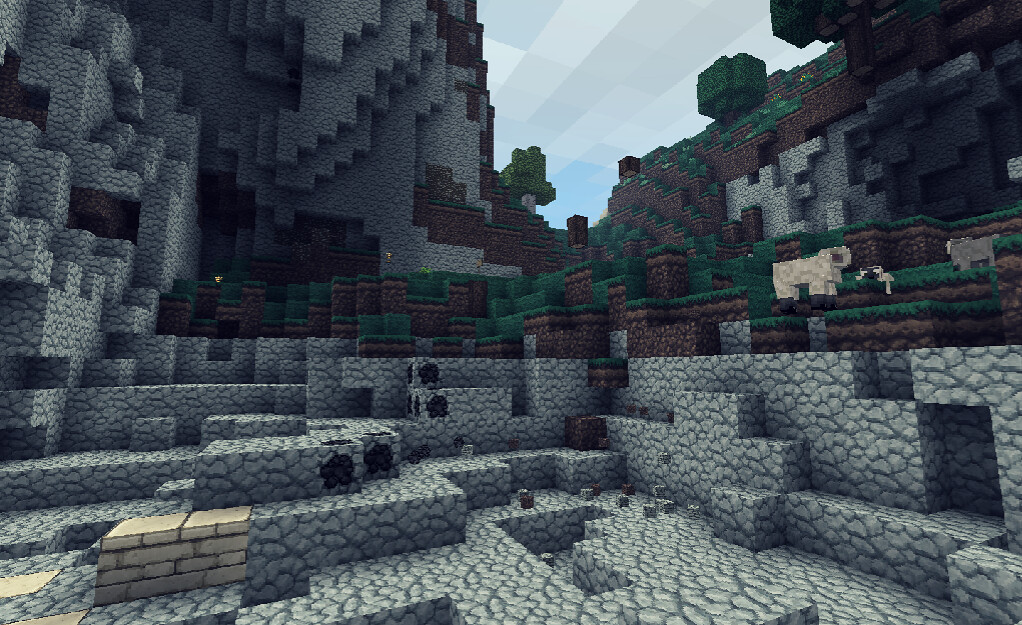This detailed visual description captures a colorful screenshot from the popular video game, Minecraft. The scene showcases the game's signature blocky aesthetic, with a diverse landscape that centralizes around pixelated dark gray blocks. Dominating the background is an imposing, towering structure made up of the same dark gray blocks, its height extending beyond the frame. 

The landscape features terraced sections composed of brown soil topped with lush green grass, creating a layered visual effect. Interspersed throughout are a number of blocky trees, seamlessly integrated into the Minecraft environment’s characteristic square style. To the far right of the terrace, a few blocky and pixelated sheep graze, embodying the game's distinctive design. The sky above is a clear blue, dotted with Minecraft's iconic blocky white clouds, completing the serene and digitally crafted vista.